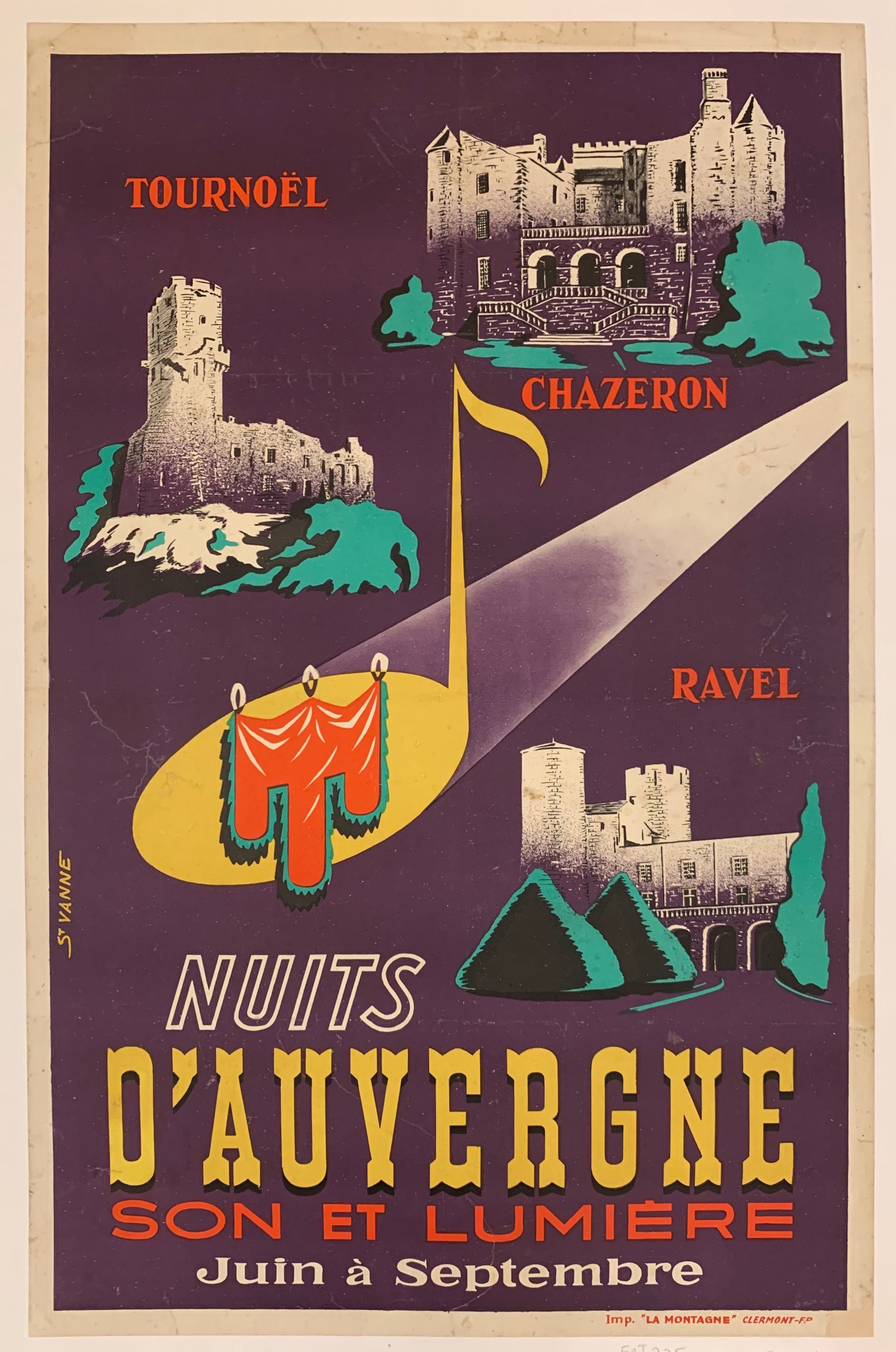The image depicts a framed poster with a light, tea-stained brown mat surrounding it. The poster itself has a slightly darker brown border and presents a detailed depiction of three castles against a plum purple background. In the upper right-hand corner, there is a black, white, and purple illustration of a castle labeled "Chazaron" in red print, accompanied by green foliage representing bushes. To the left, labeled "Tournoel" (with two dots above the 'E'), is an image of another castle perched on a cliff. Below this, a spotlight from the right highlights a figure clad in a red cloak. Towards the lower right, the poster features the third castle, identified as "Ravel" in red print, with all three castles sharing architectural elements such as arches and towers. At the bottom, the poster states "Nuits d'Auvergne Son et Lumière" in white and "Juin à Septembre" in yellow. The lower right-hand corner of the border carries the red-printed notation "IMP", followed by the phrase "La Montagne" in quotations, with "Claremont, F-P" behind it.